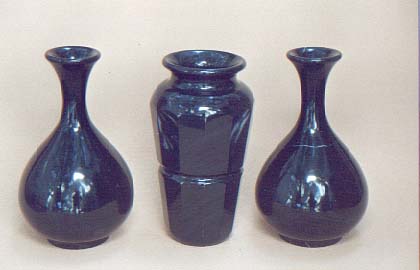In the photograph, three deep navy blue ceramic vases are arranged side-by-side against a light grey or white background, reminiscent of a store listing shoot. The two vases flanking either side are identical, featuring a design akin to garlic bulbs with a round base and a tapered, narrow neck that flares slightly at the top. These bulbous vases also display subtle white accents that blend into their glossy, shiny finish. The central vase, distinct in style, has a more robust, faceted design. It starts narrower at the base, widening towards the top, culminating in a broad, sturdy opening. This vase appears more square and solid compared to its companions. Reflections on the glossy surface, indicating a ring light and a person holding a camera, add an extra dimension to the image. A delicate print, potentially resembling small blue butterflies, adorns the two rounded vases, enhancing their intricate detail. Together, these vases present a cohesive yet varied ensemble, perfect for both decorative purposes and floral displays.